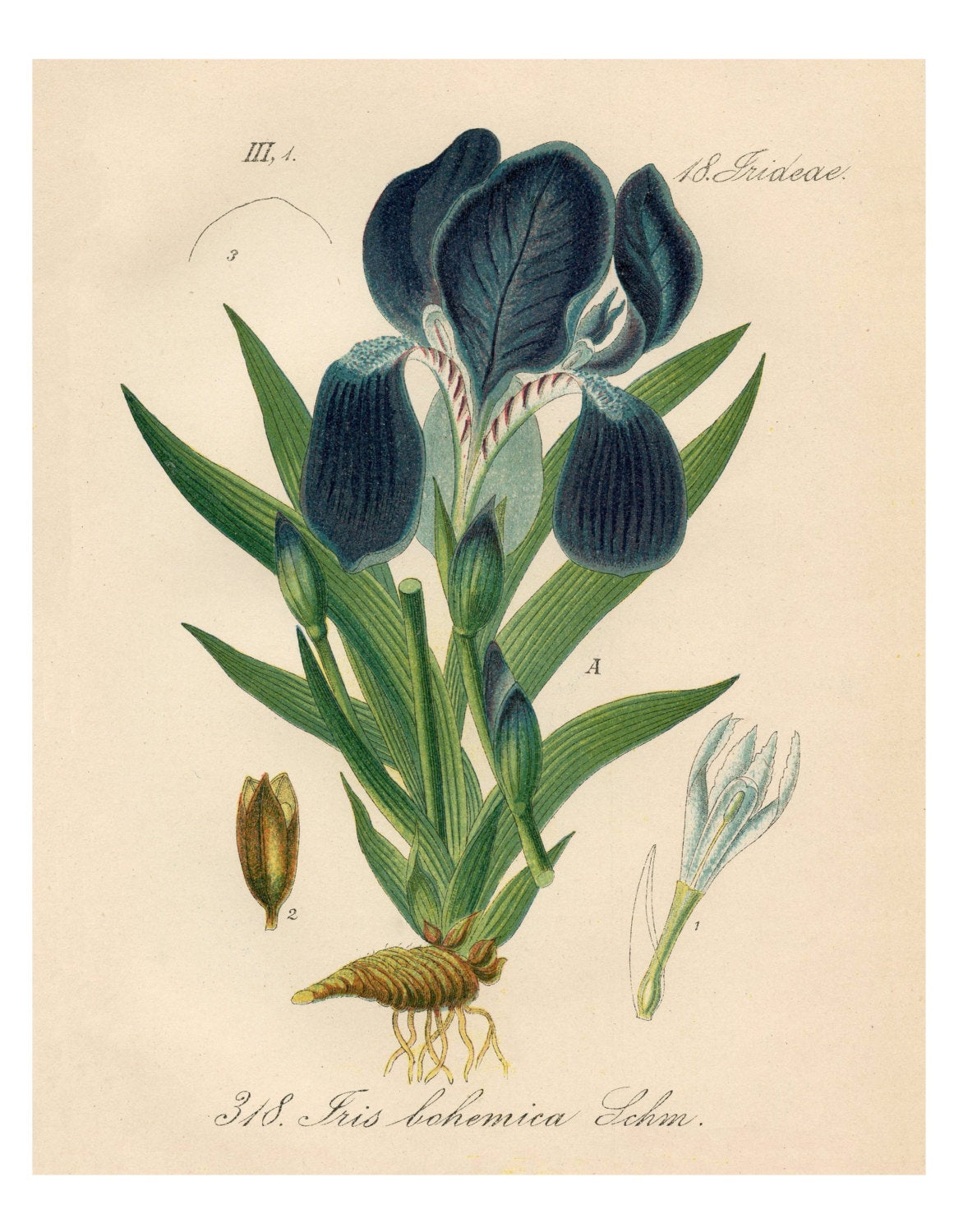This illustration features a meticulously hand-drawn flower, likely an orchid, presented on yellowed drawing paper in portrait orientation. The flower, named "Iris Bohemica John," according to the cursive subtitle at the bottom, is depicted with considerable botanical detail. Its six petals showcase a stunning gradient from midnight blue at the edges to a lighter blue towards the center, each marked with finely visible veins. A white funnel-shaped section extends from the base of the petals to the green stems, which fan outwards and support the plant. The artwork also includes detailed depictions of the plant's root structure and several green leaves radiating from the stem. Alongside the main flower are additional illustrations of a bud and seed, providing a comprehensive view of the plant's lifecycle. Roman numeral annotations scattered throughout likely refer to different parts of the flower. In the upper right corner, barely legible cursive reads "18 Fridae," adding an extra layer of historical or scientific context. The entire piece is rendered with colored pencils, enhancing its old-fashioned scientific charm.